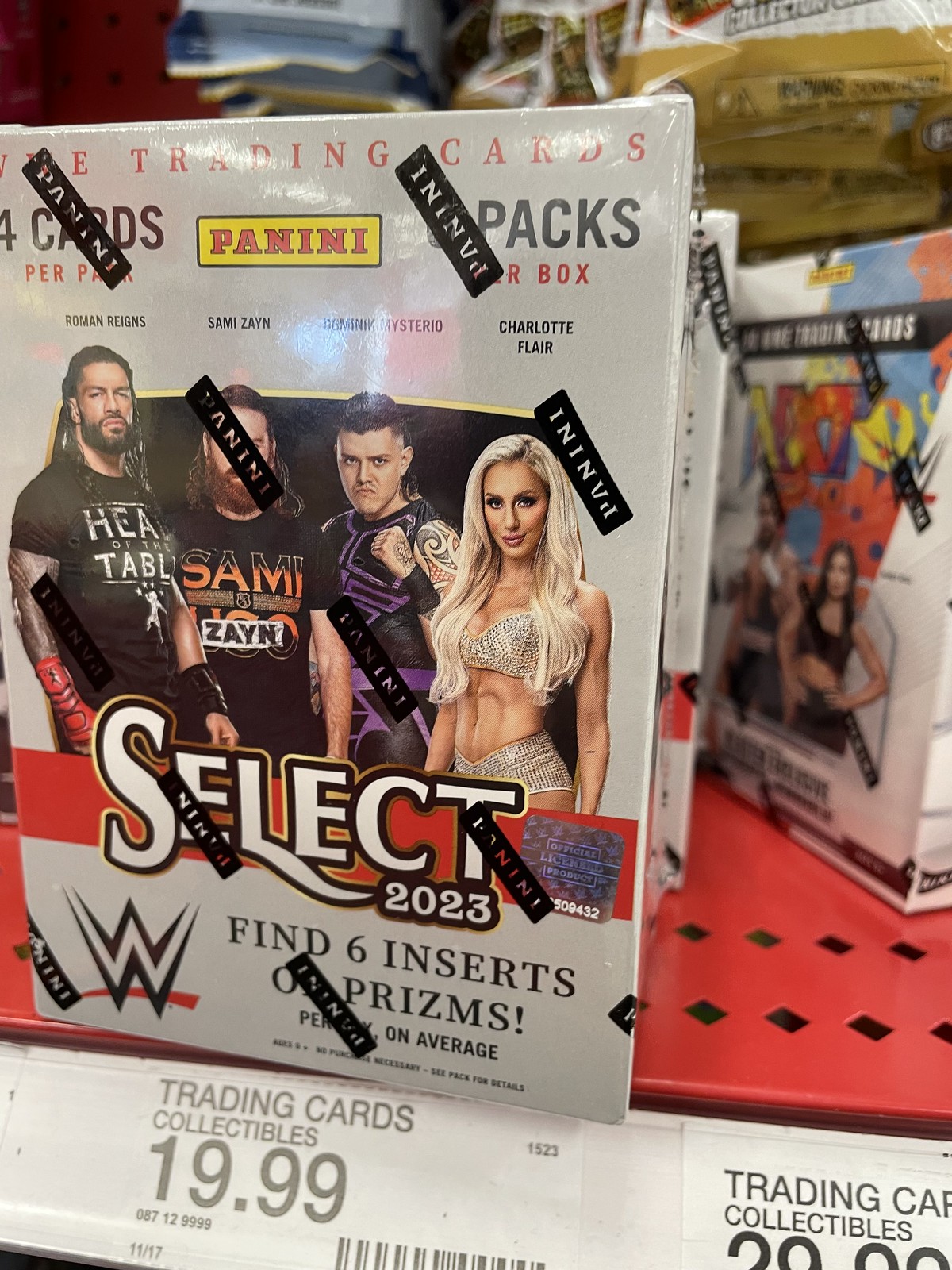This photograph was taken inside a store, likely a card trading or comic book store, given the context and products on display. The store shelf, which is red, has labels indicating pricing and product information. In the foreground is a prominently placed box of WWE trading cards, wrapped in plastic.

The box displays a clear "Panini" logo with a yellow outline and pink font. It prominently features images of four wrestlers: Roman Reigns, Sami Zayn, Dominik Mysterio, and Charlotte Flair, all wearing dark-colored clothing with graphic designs. The product is labeled with "Select 2023" below the wrestlers' images. Additionally, it mentions "Find six inserts or prisms on average".

The shelf label in front of the box reads "Trading Cards Collectibles 19.99", and several other copies or similar boxes of these trading cards are visible to the right of the main box. The combination of detailed branding, featured wrestlers, and pricing information provides a comprehensive view of this specific product in the store setting.